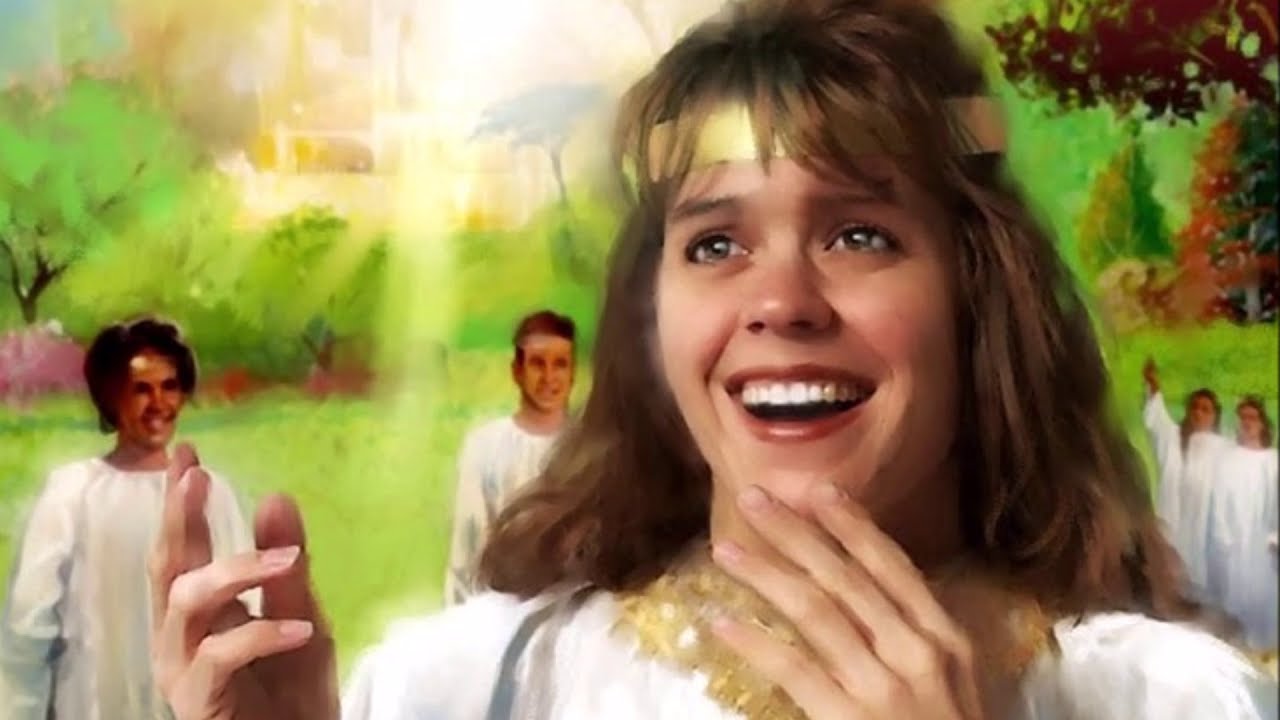The image depicts a detailed, semi-realistic scene centered around a young woman positioned slightly off-center to the right. The woman, whose image fills the frame from shoulders up, appears to be digitally rendered or painted. She has wavy, shoulder-length brown hair, a gold headband, and is adorned with an ornate gold necklace. Her attire is a white robe-like garment. She is captured mid-smile, looking slightly left of the viewer, her expressive grayish-blue eyes shining. Her hands are positioned in front of her, with the right hand near her shoulder and the left hand with two fingers touching her chin.

In the background, to her right, stand two other figures clad in white robes; one, a man with short brown hair, and the other, a woman with short dark hair. To her left, there are another man and woman, also in white robes, with the former pointing upwards. All are set against a vibrant green field adorned with trees. Behind them, the sun shines brightly, casting a noticeable glare over the scene, adding to its ethereal quality. The contrast between the crisp, photo-like depiction of the woman and the more stylized, cartoonish rendering of the background elements creates an intriguing visual dynamic, suggesting a blend of reality and fantasy.